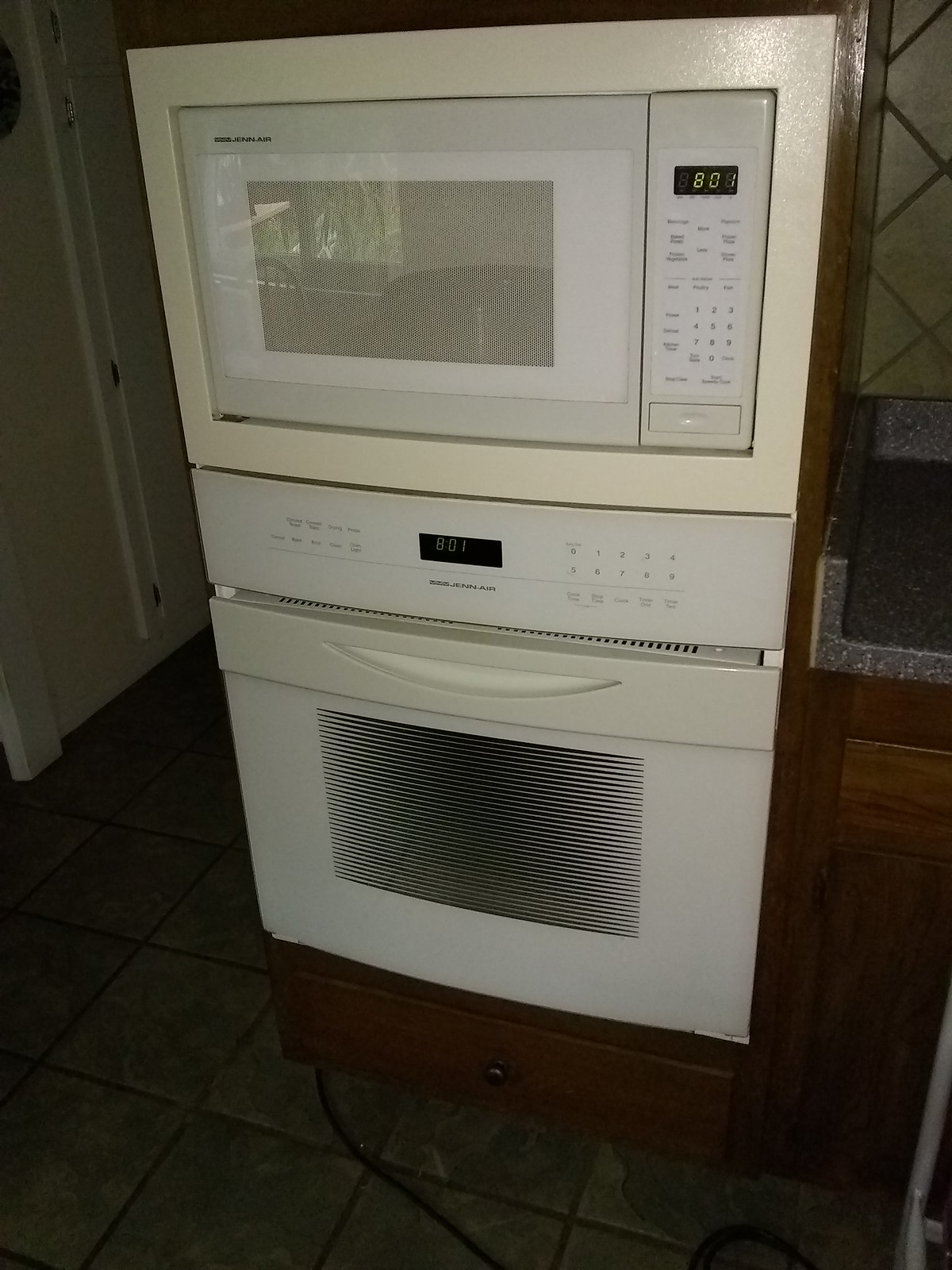This color digital photograph features a dimly lit section of a kitchen, focusing on a white two-storied microwave-oven combo built into a dark brown cupboard. The top unit, a traditional microwave with a digital display on its right showing '8:01' in green, sits above an oven-like lower unit, also with a digital clock displaying the same time. Both appliances, made of white plastic, suggest a lower quality. On the far right, a black faux-stone countertop with white specks contrasts with dark wooden cabinets below. The linoleum floor, in a dark square pattern, and a partially visible white cupboard door on the left further frame the scene.